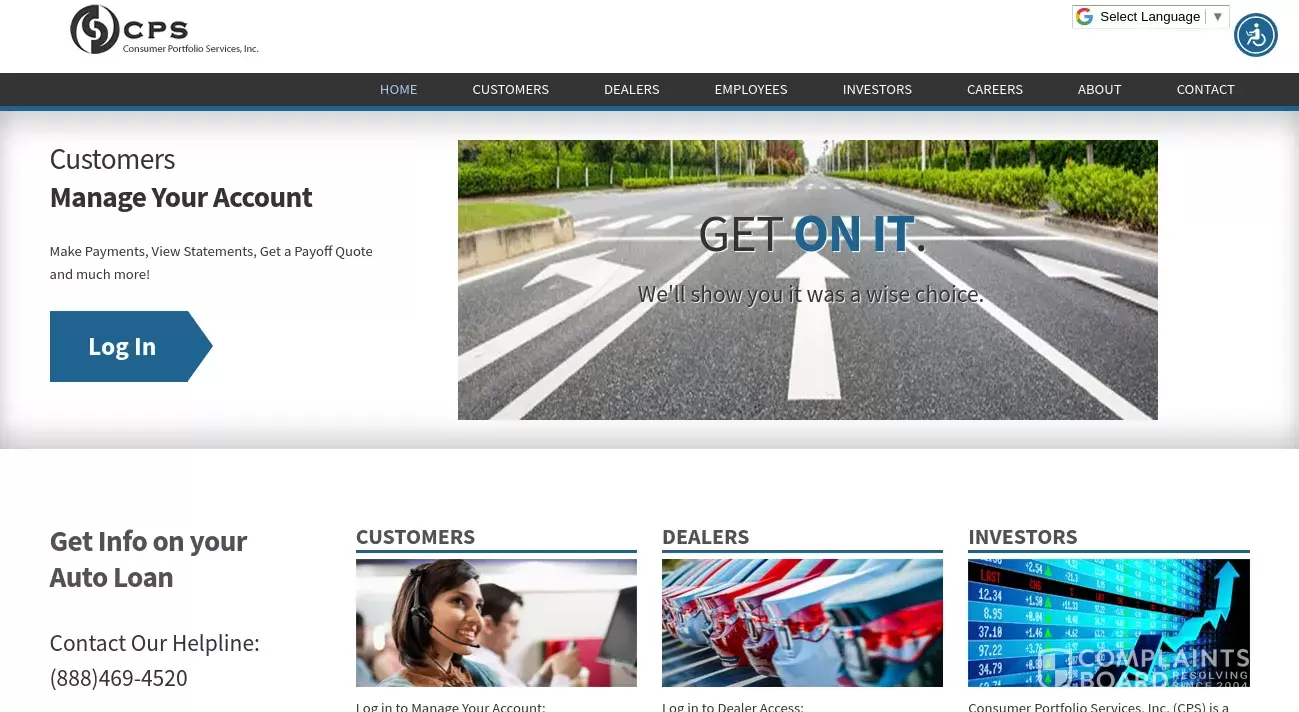This image features the homepage of the Consumer Portfolio Services, Inc. (CPS) website, adorned with a black and white logo at the top. Below the logo is the full company name, "Consumer Portfolio Services Inc." 

A prominent black banner spans the width of the page, displaying several menu options: Home (highlighted in blue), Customers, Dealers, Employees, Investors, Carriers, About, and Contact. Above this banner, a small handicap icon is followed by a blue "Select Language" link with a dropdown menu for language selection.

Dominating the center of the image is a striking road photograph, depicting an intersection with three lanes—a left-turn lane and two straight-ahead lanes. Overlain text reads "Get On It," with "Get" in black and "On" in blue. Below, a caption in white text states, "We'll show you the way."

On the left side, a section for Customers offers tools to "Manage your account" in bold text. Smaller text outlines available services: Make Payments, View Statements, Get a Payoff Quote, and much more. A right-pointing blue arrow below this section includes white text that says "Login." Further down, additional information invites users to "Get Info on your Auto Loan" and provides a customer helpline at 888-469-4520.

Three distinct menu tabs labeled Customers, Dealers, and Investors are shown at the bottom. These menus are paired with relevant images: a stock photo of a customer service representative for Customers, a picture of car bumpers in various colors for Dealers, and a snapshot of stock market numbers for Investors.